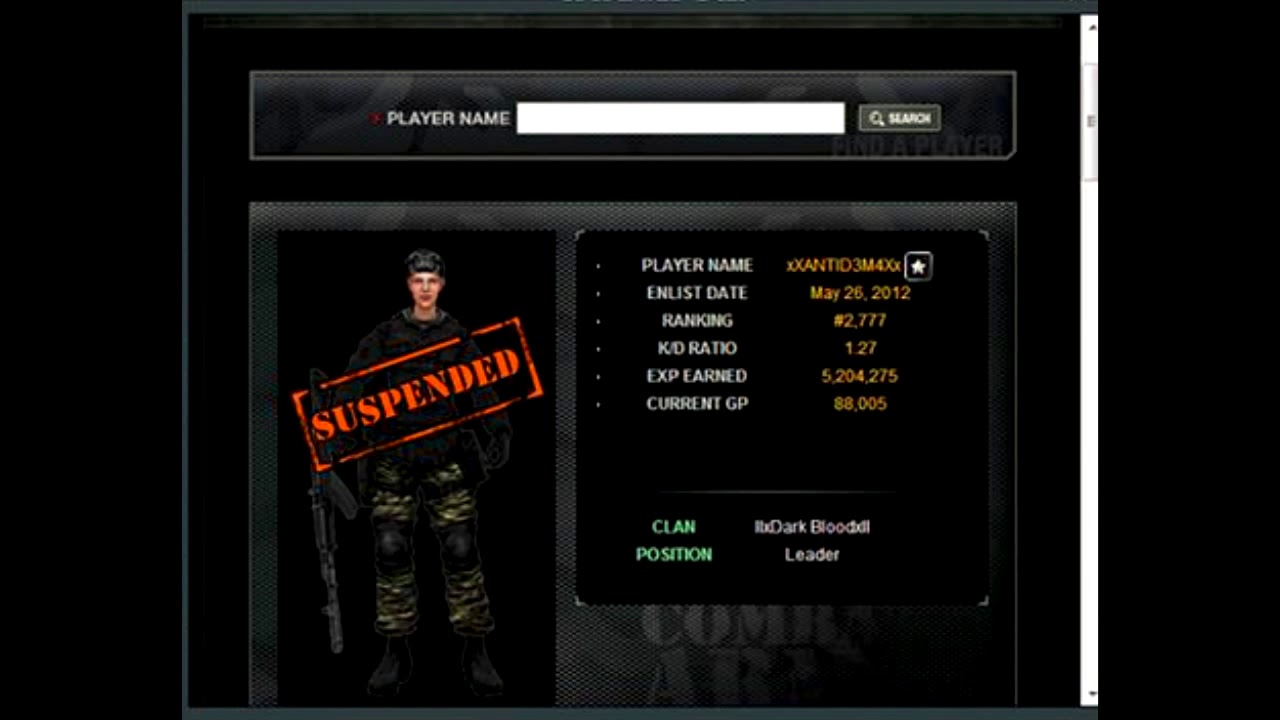The image depicts a detailed interface of a video game with a black background. At the top is a player name displayed in white, followed by a long rectangular search box with a search button next to it on the right. Central to the image is a drawing of a Caucasian male character in an army uniform, consisting of camouflage fatigues and black knee pads, holding a long gun in his right hand that touches the ground. Overlaying him is a diagonal orange rectangle labeled "suspended."

To the right of the character are detailed stats and information: beneath the header "player R name," a yellow line separates various game metrics and stats. In capital white print, "Enlist Date" is accompanied by "May 26, 2012" in yellow. Other stats include "Ranking" at 2,777, "K/D Ratio" at 127, "EXP Earned" at 5,204,275, and "Current GP" at 8,005. At the bottom of these details, in blue or green uppercase writing, "Clan" is followed by "Dark Blood" and "Position" in green, with "Leader" in white. A scroll bar on the right indicates that this interface is displayed on a tablet or desktop. The entire layout conveys a tactical and military-themed video game screen.